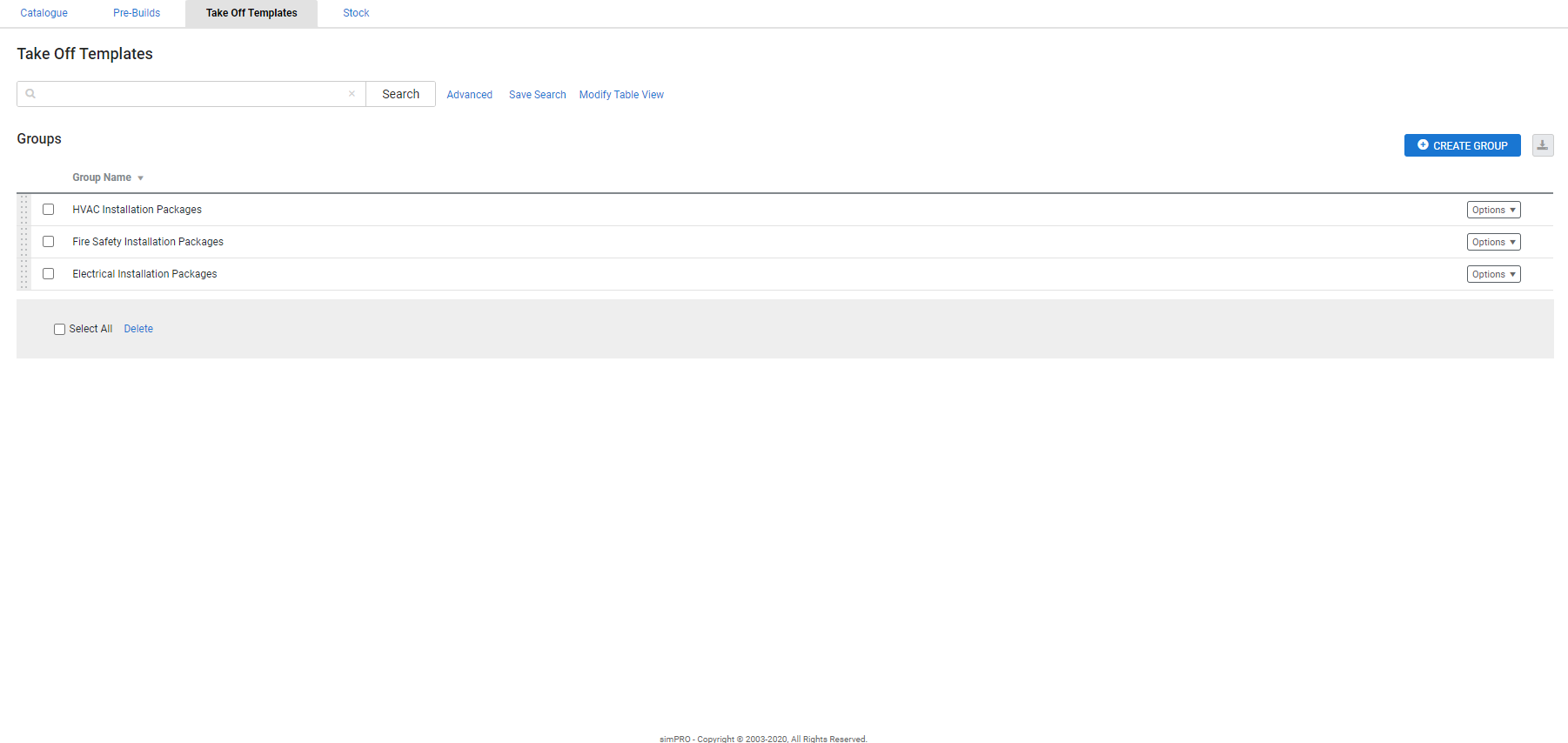The web page features a clean, white background and is organized with a structured layout for easy navigation. At the top, the page includes a navigational menu with the following options in blue text: "Catalog," "Pre-Builds," and "Stock." Additionally, there is a gray rectangle with bold black text that reads "Take Off Templates."

Below the navigation menu, "Take Off Templates" appears again, followed by a search bar labeled with the word "Search." Adjacent to the search bar are several options in blue text: "Advanced," "Save Search," "Modify Track," and "Table View."

On the left side of the page, under a section labeled "Groups," there is a rectangle box featuring a list of installation packages. At the top, this box has a header titled "Group Name," and below it are the following groups:

- HVAC Installation Packages
- Fire Safety Installation Packages
- Electrical Installation Packages

Each group is marked with a white, square-shaped bullet point.

To the right side, in line with each package group, there are options for "Create Group" and an "Options" button with a black down-arrow, indicating a drop-down menu is available.

The bottom of the page concludes with a gray bar, rounding out the structured and user-friendly design.